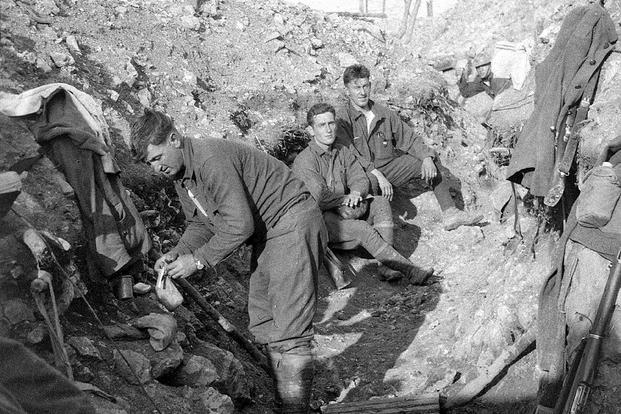This black-and-white photograph, likely a historical wartime image, captures a moment of respite for four soldiers in a trench surrounded by rubble and rocks. Three of the men are positioned centrally. The man closest to the camera, on the left, is bent over, appearing to search through a bag or tend to some clothing items and a canteen at his feet. Behind him, two soldiers are seated; one is cross-legged with his hand on his knee, wearing a military jacket with a collar, and gazes directly at the camera. The other, sitting with one leg crossed over the other, also seems to be taking a break. A fourth soldier is visible in the background, standing and possibly holding or adjusting something that isn’t entirely clear. Personal items, including guns, canteens, and additional clothing, are strewn about or draped on the rocks lining the trench. All the men have short, military-cut hair, and their fair skin suggests they are either American or European. The atmosphere is one of weary respite amidst the harsh, rocky environment of war.